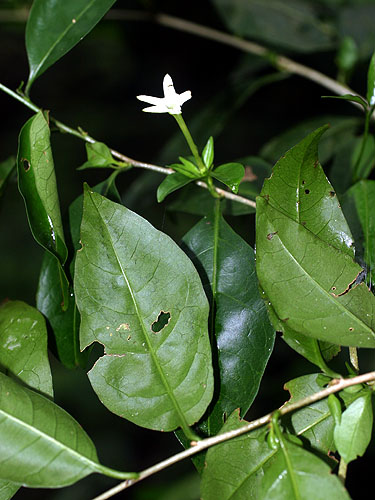A close-up image captures a delicate scene featuring dense foliage of a vine plant. The focus centers on a light tan twig around which a vine is climbing. The vine is adorned with dark green leaves, many of which bear holes or chunks, likely from being eaten by bugs. Some of the leaves feature brown outlines around the damaged sections. Among the leaves, a small white flower with five petals blooms at the top of the vine, resembled a star shape. The main leaf at the center of the image exhibits a large perforation on the left and a hole on the right, highlighting the close-up details. The background of the image is blurred and black, giving the impression that the photo might have been taken at night, emphasizing the sharpness of the flower and foliage in the foreground. Overall, the image captures the intricate details of the vine and its fragile ecosystem.